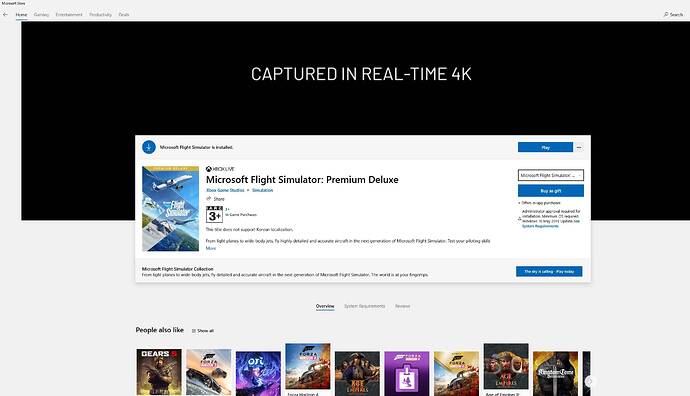Here is the cleaned-up and detailed caption for the image:

---

This image is a computer screenshot with a light gray background. In the upper left corner, there is some bolded black text that is unreadable. About two lines below, a menu bar stretches horizontally across the screen, containing five unreadable black words. At the far right edge of this menu bar, there is a single black word. Directly beneath this, there's a large black horizontal rectangle with the phrase "CAPTURED IN REAL-TIME 4K" written in bold white capital letters near the top.

Approximately four lines below the black rectangle, a large white square occupies the central portion of the screen. In the upper left of this square, a blue circle with a white downward-pointing arrow appears, accompanied by some unreadable black text to the right. Towards the right side of the square, there is a blue rectangle with an opaque white word inside, also unreadable.

Beneath this area, to the left, is an image featuring a jet soaring through a blue sky with some distinct blue, white, and brown rectangular shapes at the bottom. To the right of this image, the text "Microsoft Flight Simulator: Premium Deluxe" is prominently displayed in black. A descriptive text block follows underneath this title.

On the right-hand side of the screenshot, there are several boxes. The top box is outlined in gray and contains some text, followed by a blue rectangle with white text inside it, both of which are unreadable. At the very bottom of the image, a series of horizontal squares depict either books or movies, spanning across the entire width of the screen.

---

This enhanced caption aims to provide a comprehensive and clear description of the screenshot and its elements.